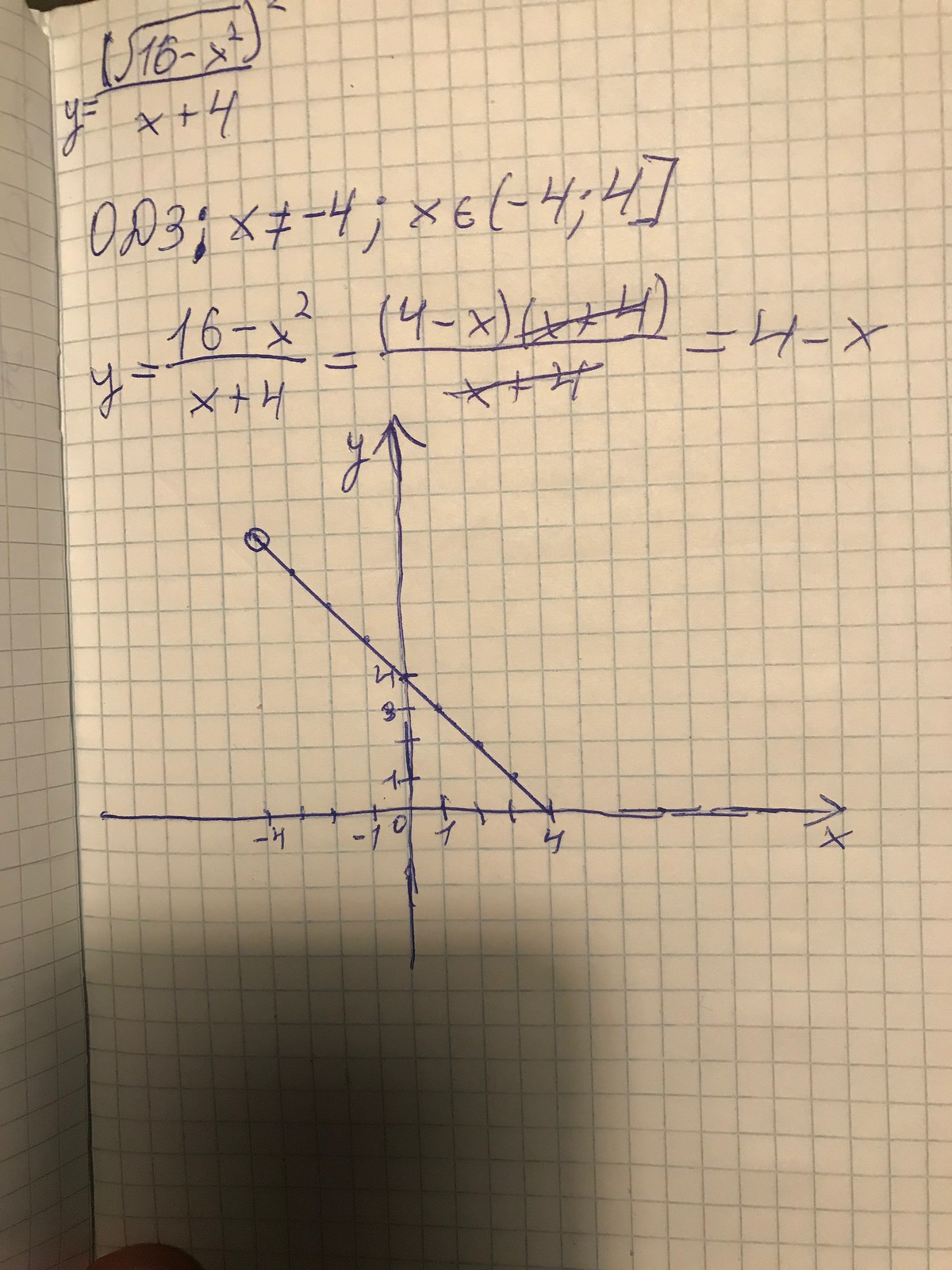In the image, a complex mathematical equation is meticulously written out on a sheet of graph paper, filling the entire frame with no other background elements visible. The equation initiates in the upper-left corner with "Y =", and is followed by a classic division format. The numerator of this fraction features the expression "(16 - X²)²", where both the outer exponent and the X exponent are 2. The denominator is a simple "X + 4".

Below this initial setup, there's another row containing the elements: "0, possibly a P, 3; X ∥ -4; times E", and then the range "( -4, 4 )" squared yet within parentheses.

Further down, the equation is rewritten: "Y = 16 - X² / (X + 4)", equating to "(4 - X)" with "(X + 4)" canceled out line by line. The repeated division expression is distinctly marked through multiple crossings-out: "(X + 4)" is negated, simplifying to "Y = 4 - X" after specific cancelations.

On the lower section of the paper, a coordinate graph stands out prominently, featuring a vertical arrow marked with "Y" at the top and a horizontal arrow marked with "X" at the right end. A diagonal line extends across the graph, dotted at each intersecting point on the graph paper. Along the vertical axis, marks represent values 1, 3, 4, and notably exclude 2. Horizontally, markings include "-4, -1, 0, 1", and "4".

This carefully drawn arrangement highlights the effort and precision involved in solving and illustrating the equation, reflecting both the process of mathematical manipulation and the graphical representation of the solution.